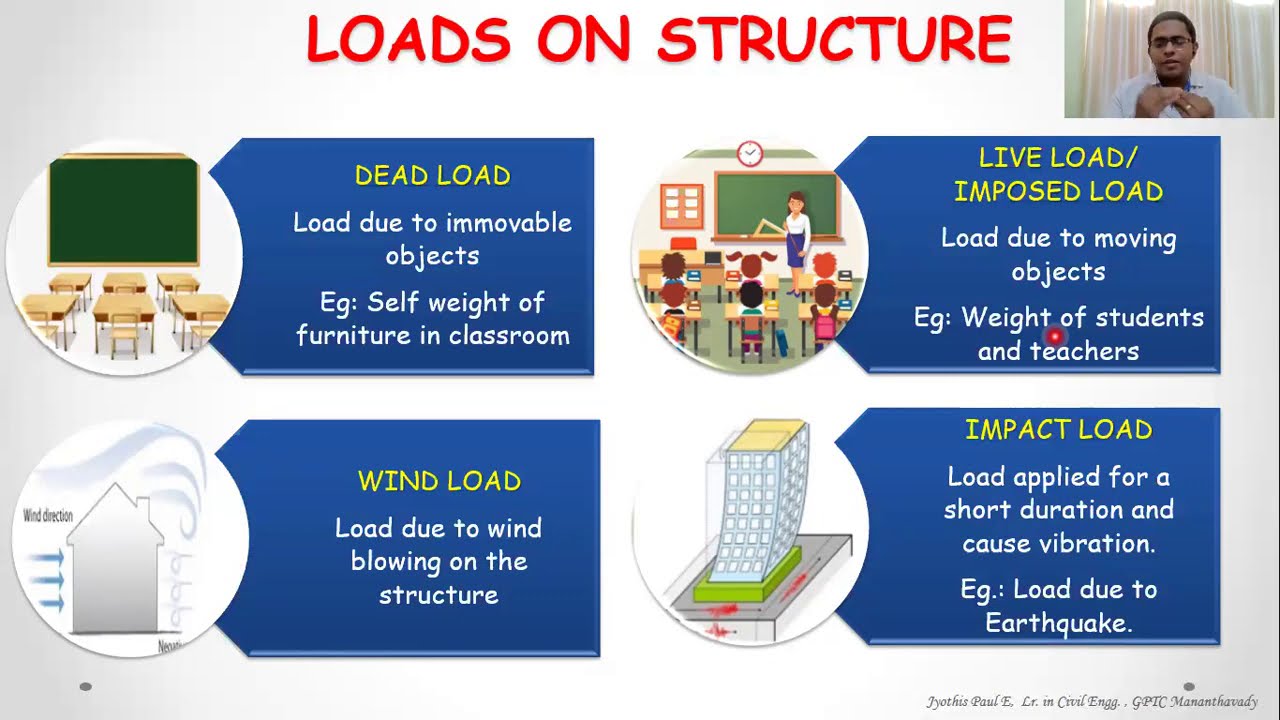The image depicts a screenshot of an online civil engineering lecture titled "LOADS ON STRUCTURE." The slide, with a gray-white background, is detailed with four sections explaining different types of structural loads. In the top-right corner, a man with short black hair and black-rimmed glasses, named Jayothis Paul E., a lecturer in Civil Engineering at GPTC, Mananavati, is live-streaming. He is standing in front of moss green curtains, wearing a light blue collared shirt. Jayothis appears to be gesturing with his hands clasped, showcasing a ring on his right hand. The four sections of the slide are as follows:

1. **Dead Load**: Illustrated with an image of a classroom, it explains that this load is due to immovable objects, such as the self-weight of furniture in the classroom.
2. **Live Load/Imposed Load**: Featuring a classroom scene with students and a teacher, it describes this load as resulting from moving objects, like the weight of students and teachers.
3. **Wind Load**: Depicted with an image of a house subject to wind forces, it details that this load is due to wind blowing on the structure.
4. **Impact Load**: Shown with a building during an earthquake, it notes that this load is applied for a short duration and causes vibration, exemplified by earthquake forces.

Additionally, a possible laser pointer marks the section on Live Load/Imposed Load. The lecture slide is methodically laid out with each section containing an icon, subtitle, and explanatory text.